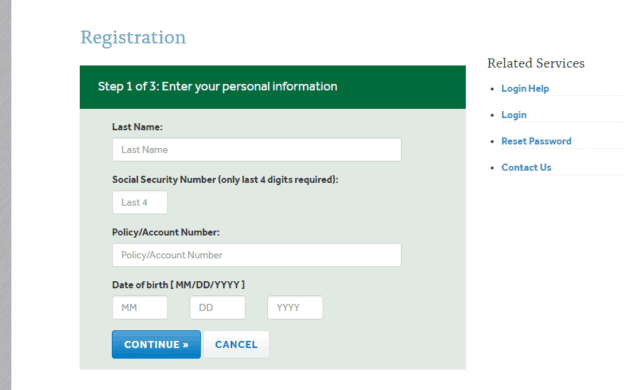The image depicts a registration screen set against a light gray background. The screen heading reads "Registration". Below, there is a green rectangle with the text "Step 1 of 3: Enter your personal information" written in white. The form contains fields labeled "Last Name," "Social Security Number," "Policy Account Number," and "Date of Birth," each accompanied by white rectangles where users can input their information. At the bottom of the form, there is a blue rectangle with the word "Continue," and to its right, a white rectangle labeled "Cancel" in blue text.

On the left side of the image, a vertical gray bar runs from top to bottom. On the right side of this bar, the text "Related Services" appears, followed by four blue clickable options: "Login Help," "Login," "Reset Password," and "Contact Us."